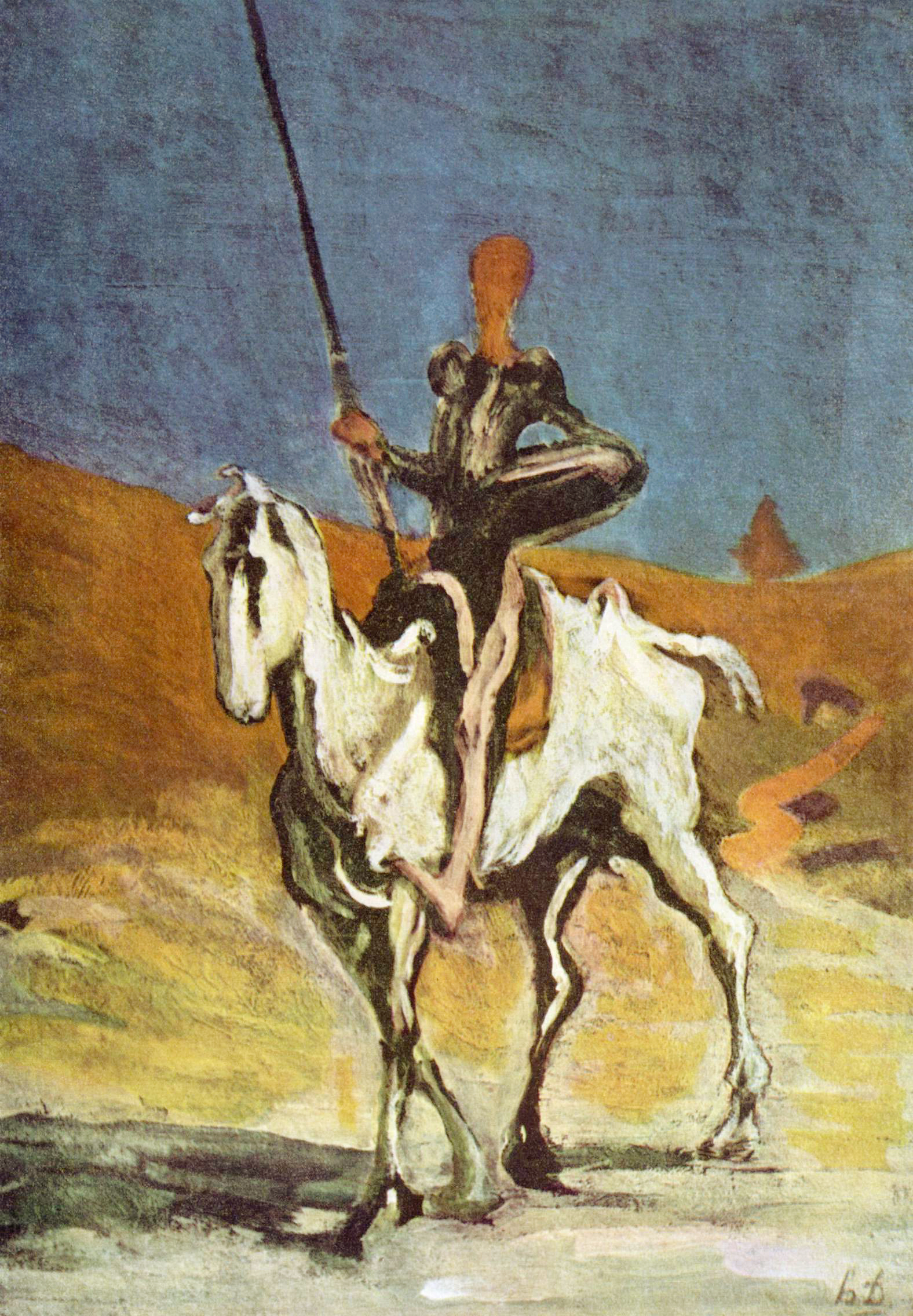This image is a photograph of a slightly surreal painting depicting a soldier riding a white horse through a desert-like landscape. The boundaries of the person and the horse are blurred and wavy, with muted tones dominating the entire scene. The soldier, who appears to be holding a large sword and possibly a helmet at their side, wears a black bodysuit and has an orange face with no distinguishable features. The surrealism of the painting renders the rider faceless and the intricate details difficult to discern. The horse features black marks around its eyes, and the landscape adds to the mystique with a cobalt blue sky tinged with gray and a sprawling brown desert that transitions into yellow and white sands. The composition includes a small tree, a path-like structure, and what appears to be a black log in the foreground, all drawn with a lack of distinctness. The horse and rider cast a black shadow on the ground, enhancing the slightly dreamlike, ethereal quality of the scene.